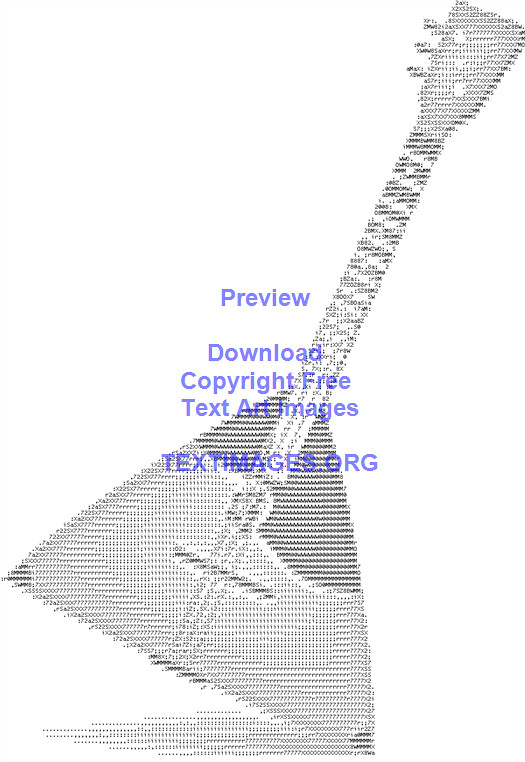The image depicts a string instrument resembling a guitar but with a distinctive triangular body and only three strings and tuning knobs. This guitar is portrayed using computer-generated ASCII art, where various symbols, numbers, and letters are meticulously arranged to form the detailed shape of the instrument. The neck of the guitar angles towards the top right corner of the image. Superimposed on the artwork, in a blue font, are the words "Preview" and "Download," followed by "Copyright Free Text Art Images." Beneath this, in bold capitalized letters, is the website "TextImages.org". The background is stark white, providing a sharp contrast to the black ASCII art of the instrument.